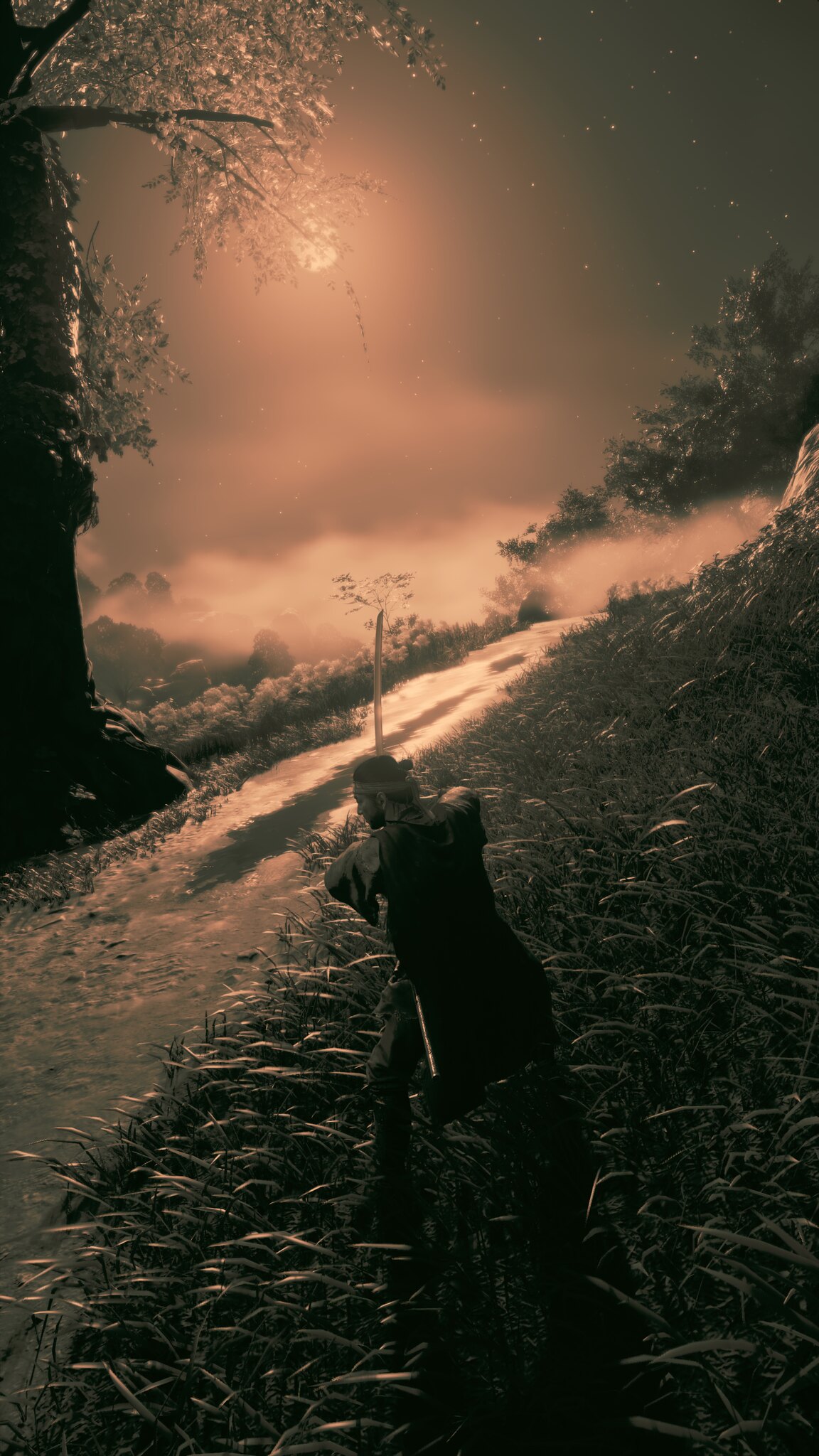The image depicts a young warrior immersed in a fantastical scene reminiscent of both a movie still and a video game screenshot. The setting is a dark, eerie forest, cloaked in a dense fog that blankets the ground and path before him. Bathed in a burnt sepia tone, the entire image is suffused with an orange hue, suggesting either dawn or dusk. 

The warrior stands in tall, knee-length grass, his posture poised and ready for combat. Clad in a long, dark cloak that reaches his knees, he also dons a bandana wrapped around his head. A sword is sheathed at his left hip, while another is gripped firmly in his outstretched arms, angled in front of him, as if preparing to strike. His stance is one leg forward, hinting at imminent action.

To his left, a dirt path meanders off into the background, interrupted by a large tree with sprawling branches. One branch arcs downward, nearly touching a small orange circle in the sky, presumably the sun. This sun casts a warm, golden glow that permeates the sky, mingling with rolling clouds and a thick mist that envelops the forest floor, giving the scene an almost otherworldly ambiance. 

In the background, the path straightens and then curves out of sight, suggesting the hidden dangers or adventures that lie ahead. Off to the top right of the image, the dark sky is speckled with stars, and the silhouette of another tree can be discerned, adding to the mystique. The entire composition—complete with its dark colors, dramatic lighting, and detailed textures—evokes a sense of suspense and anticipation as the warrior stands ready to face whatever challenges await in this enigmatic, sepia-toned world.